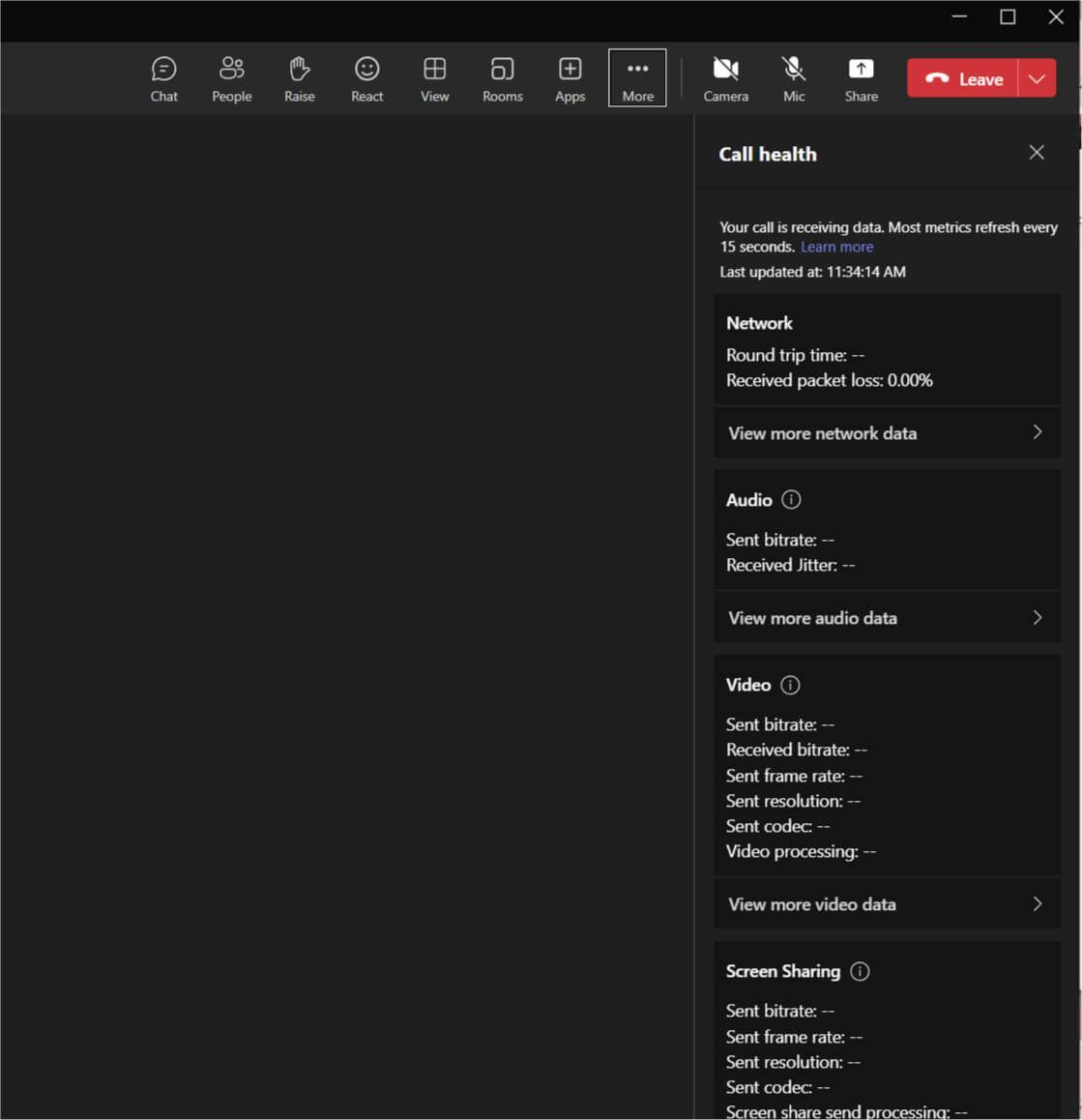This image displays the interface of a communication software similar to Zoom or Skype, but not one that is immediately recognizable. The top of the interface features a black strip, and directly below it is a dark grey strip containing various white icons from left to right: 

- A speech bubble labeled "Chat"
- Two people icons labeled "People"
- A hand icon labeled "Raise"
- A smiley face labeled "React"
- A grid of four blocks labeled "View"
- A small square in front of a larger square labeled "Rooms"
- A square with a plus sign inside labeled "Apps"
- Three dots in a line labeled "More," which is highlighted with a square white outline.

Further along the strip to the right:
- A camera icon with a line through it, indicating that the camera is turned off
- A microphone icon with a line through it, indicating that the microphone is turned off
- A white rectangle with a black up arrow labeled "Share"
- A red tab with a white telephone icon labeled "Leave", accompanied by a drop-down arrow.

The central part of the screen is mostly empty, suggesting that no current video call or meeting is active. To the right of this empty space, a section labeled "Call Health" provides data on the call's status, stating that "Your call is receiving data, most metrics refresh every 15 seconds, last updated at 11:34:14 AM". However, given that there is no active call, this section currently shows no activity.

Overall, the interface is designed for organizing and managing a virtual meeting, complete with options for communication, interaction, view settings, app integration, and call management.